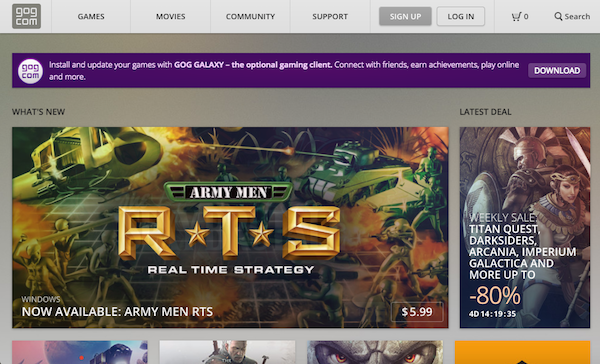The image is a horizontally rectangular partial screenshot from GOG.com, visible from the site’s upper sections but cutting off before the lower portion. The upper-left corner features the GOG.com logo, confirming the website. The top banner is light gray and includes multiple navigation options from left to right: 'Games', 'Movies', 'Community Support', followed by 'Sign Up' and 'Login' buttons. There is also a shopping cart icon displaying zero items, and a search option.

Beneath this, there is a dark purple banner with the circular GOG.com logo. The banner’s white text advertises: "Install and update your games with GOG Galaxy, the optional gaming client. Connect with friends, earn achievements, play online, and more." To the far right of this banner is a light purple download button.

Following this banner, a large, horizontally rectangular image under the section titled 'What's New' promotes "Army Men RTS Real Time Strategy," indicating it is now available for $5.99. To the right of this large image is a vertically rectangular ad for the Weekly Sale, offering discounts up to 80% on titles such as Titan Quest, Darksiders, Arcania, Imperium Galactica, and more.